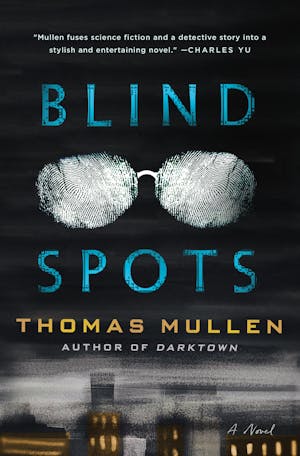This image shows the cover of a book titled "Blind Spots" by Thomas Mullen. The background transitions from black at the top to gray in the middle and white at the bottom. At the very top, a testimonial in white text reads, "Mullen fuses science fiction and a detective story into a stylish and entertaining novel," attributed to Charles Yu. Below this quote, the title "Blind Spots" is prominently displayed in large blue letters, with a drawing of glasses—showing only the frames and nose piece—strategically placed between the words "Blind" and "Spots." Under the title, Thomas Mullen's name appears in yellow text, followed by the line "author of Dark Town" in white. At the bottom of the cover, a subtle, somewhat blurry illustration of a cityscape with several buildings is visible, adding a final touch to this intriguing and stylish design. The phrase "a novel" is inscribed in white cursive text in the bottom right corner.